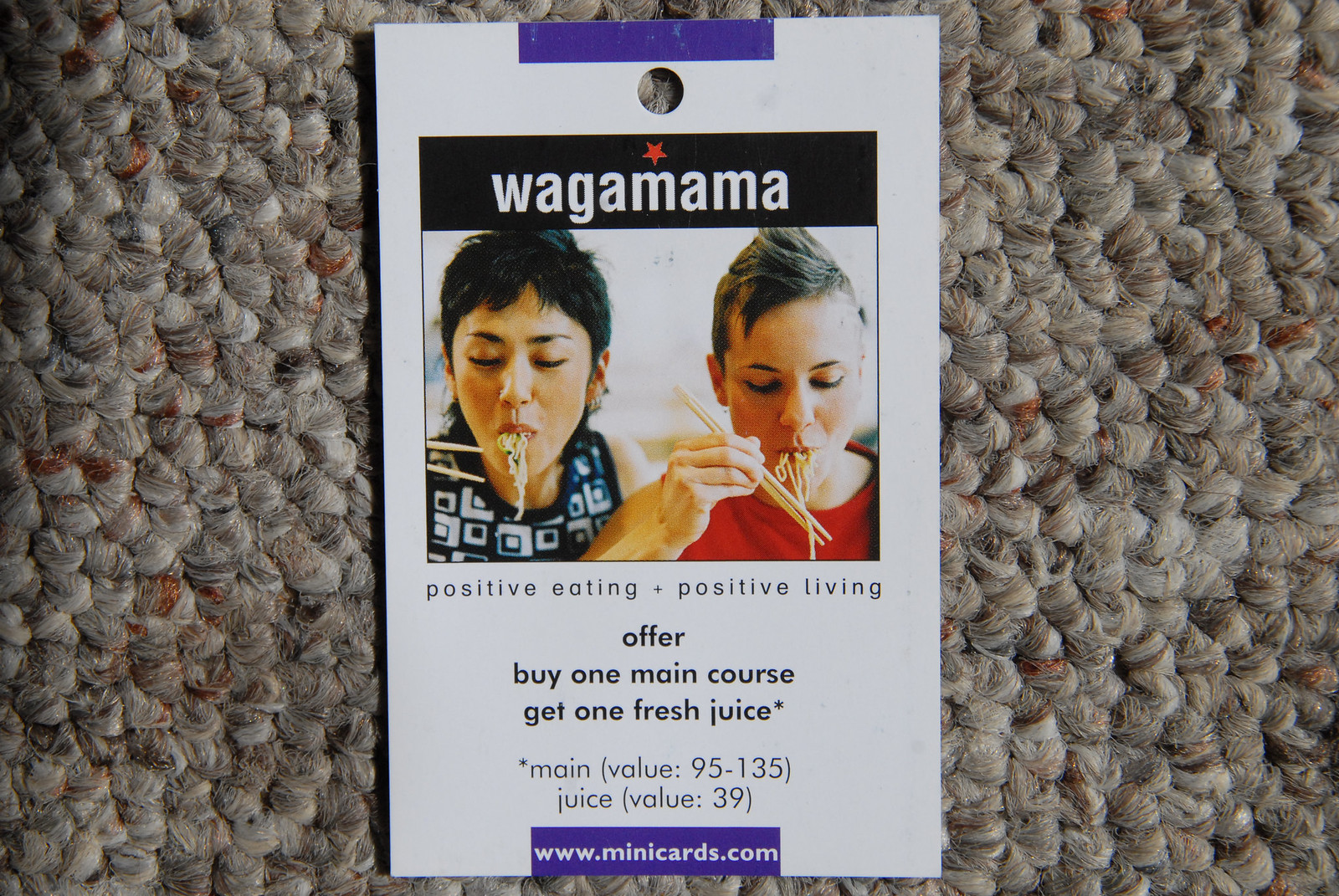The image features a tall, rectangular coupon placed on a gray, bumpy rug that appears to be woven from various colored threads, including brown and black. The coupon is white and has a purple rectangle at the top and bottom, with a hole punched below the top stripe. The top of the coupon displays a small square image of two women with short hair eating noodles with chopsticks; one has dark brown or black hair and a black shirt with white squares, while the other has light brown hair and wears a red shirt. Above them, a black rectangle contains the text "Wagamama" in white font, with a red five-pointed star. Below the image, it reads "positive eating + positive living" in black font, followed by "Offer: buy one main course, get one fresh juice." The value of the main course ranges from $95 to $135, and the juice is valued at $39. The bottom purple stripe features the website "www.minicards.com."